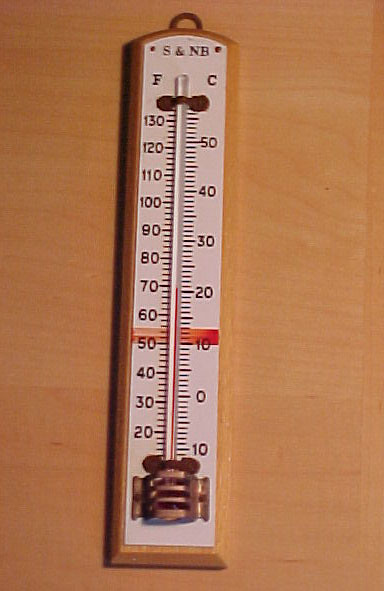The image depicts a single item, which is a classic thermometer, placed on a light blonde wooden tabletop. The smooth surface of the tabletop features subtle, slightly darker grain lines providing minimal texture. The thermometer, which could also be hung on a wall, is crafted from slightly darker wood and lies flat on the tabletop. 

The thermometer's display is predominantly white, showcasing clear black hash marks that indicate temperature readings. On the left-hand side, the Fahrenheit scale ranges from 0 to 130 degrees, with markings at every 10-degree increment. On the right-hand side, the Celsius scale ranges from -10 to 50 degrees, with similar 10-degree separations. 

A slender glass tube filled with red liquid runs vertically down the center of the thermometer, secured in place by metallic fastenings. The secure points include bent metal brackets, which have a rustic brown hue, and a firm metal clip at the bottom to ensure the thermometer's stability and accuracy. The meticulous craftsmanship and classic design make this thermometer not just a functional tool but also an aesthetically pleasing object.